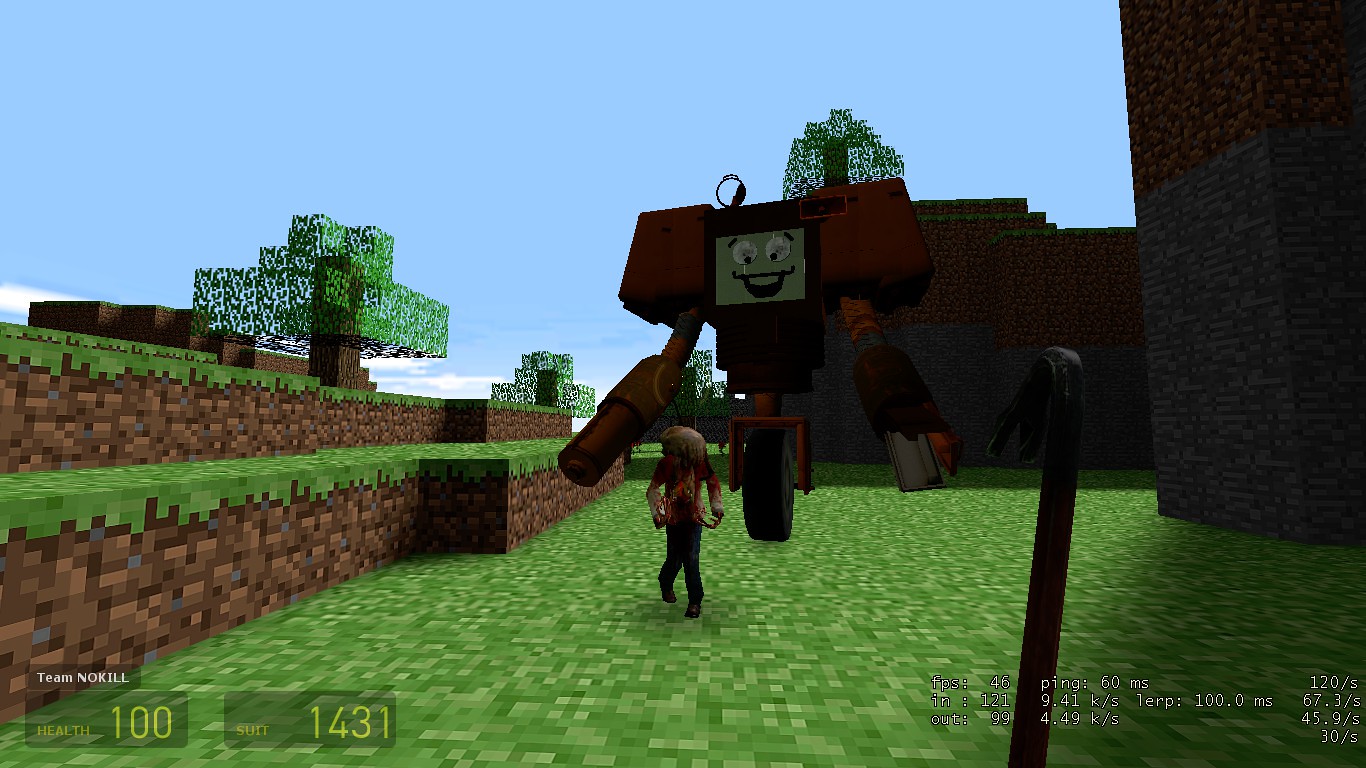Screenshot of a vibrant Minecraft landscape, capturing a player in motion. The scene is filled with iconic pixelated blocks: brown dirt blocks topped with lush green grass prominently featured. This environment evokes memories of creative gameplay, reminiscent of cherished moments building virtual worlds. The expansive land showcases rich greenery, with an assortment of trees scattered throughout, including a notably large one standing tall. To the left, two smaller trees are visible adjacent to a brown building, partially obscured by the natural foliage.

At the foreground, a character's avatar faces away, engaging with a large robotic figure centered in the image. This robot appears to be interacting with the player's avatar, though specific details about the avatar's appearance remain indistinct. On the right side, a towering dark wall frames the scene, contrasting sharply with the bright terrain. The bottom left corner includes the text "Team Norel," suggesting the involvement or identification of the player within a specific group or community in the game.